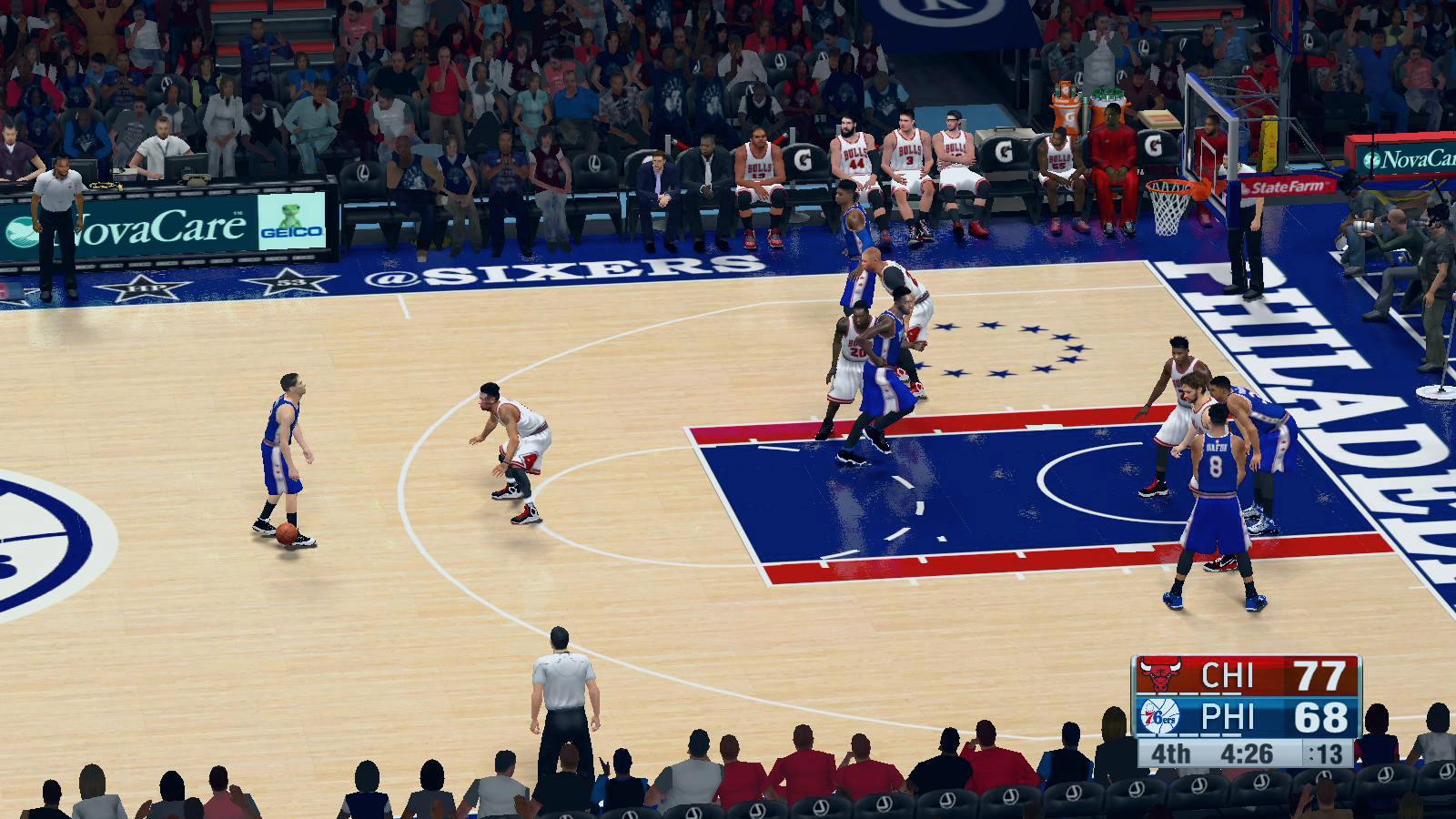This image captures a highly realistic scene from a video game of an ongoing basketball match between the Chicago Bulls and the Philadelphia 76ers. The setting is the Philadelphia home court, clearly indicated by the court's markings. As the game progresses into the fourth quarter, the Bulls are leading with a score of 77 to 68, and there are exactly 4 minutes and 26 seconds left on the game clock. The shot clock indicates that there are 13 seconds remaining for the offensive play. The Chicago Bulls bench is visible in the upper portion of the image, with five players seated on Gatorade-branded chairs. One player stands out in a red track jersey, perhaps due to his distinctive attire compared to his teammates. The level of detail, from the players' expressions to the branding on the seats, gives the impression of an almost photo-realistic depiction.